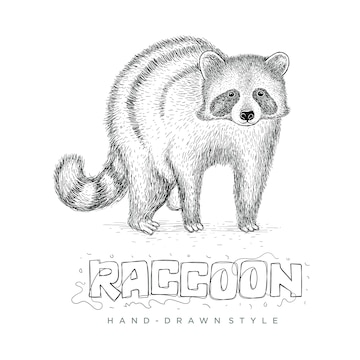The image is a detailed black and white hand-drawn depiction of a raccoon. The raccoon is facing forward, with its body slightly turned to the right. It has a very furry body, rounded ears, and long legs. The front paws are positioned out in front, with the back right foot visible next to the front right foot, while the back left foot is out of view. The raccoon's face has distinctive dark shading around the eyes, a black nose, and the top of its head is gray. Its tail, which curves slightly upwards, features prominent black stripes. The word "RACCOON" in outlined capital letters appears at the bottom of the drawing. Below that, in a smaller print that may be blue or gray, the phrase "hand-drawn style" is inscribed. The entire illustration is set against a white background.